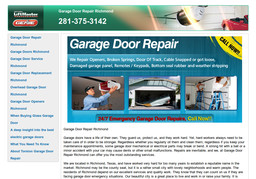A detailed screenshot of a garage door repair webpage. The top menu banner features a gradient that fades from green into an indistinct photographic image, likely of the inside of a garage. At the upper left-hand corner, a business logo is visible. Within the green section of the banner, white text prominently displays "Garage Door Repair" followed by a word and phone number: "281-375-3142". A left-hand vertical menu against a light gray background showcases blue text for 18 options, although the text is blurry and unreadable. 

Further down, a blue rectangular inset contains white text that reads "Garage Door Repair". In the upper right-hand corner, a bold yellow graphic with black text urges viewers to "Call Now". Beneath this, two lines of white text appear, though they too are challenging to read. Below these, three photographs depict a worker actively repairing a broken garage door. Directly underneath these images, in bold red text, it states "24-7 Emergency Garage Door Repair," accompanied by another "Call Now" prompt in yellow text.